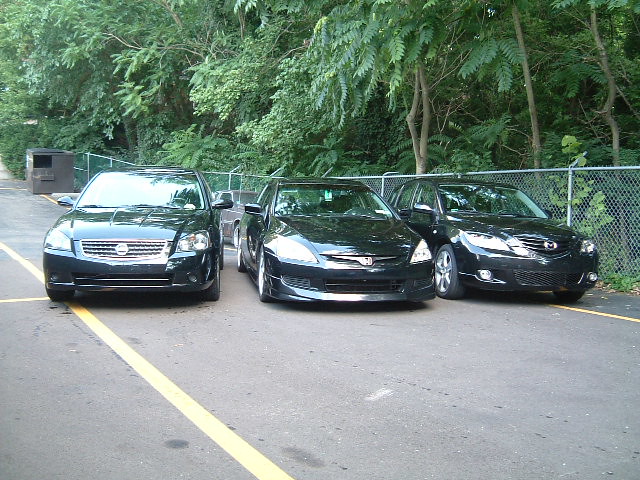In this image, three shiny, dark-colored sedans—likely black—are parked closely together at varying angles along a paved road that appears to be going uphill. The cars are positioned side by side, almost as if on display, and are marked by their distinct, albeit unidentifiable, front grilles indicating they are from different brands; one seems to be a Honda. Yellow lines segregate their parking spaces. Behind these cars stands a tall chain-link fence, which separates the road from a dense green forest, giving the impression of a jungle. In the background, a fourth car and a small gray container with a hole are visible. The scene is illuminated by light coming from the left, creating a reflective glare on the vehicles. Scattered green shrubs and trees further emphasize the lush background, and there is a hint of a small building in the far distance.